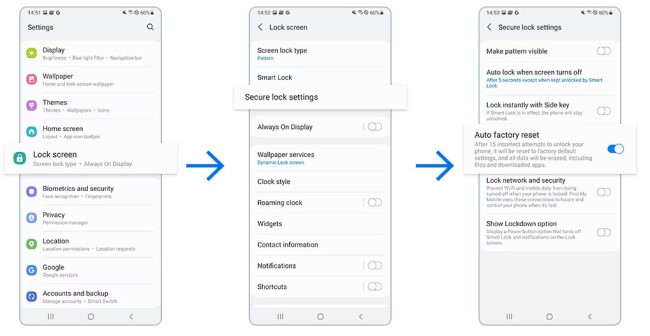This image showcases three smartphone screens side-by-side, each displaying different sections of the phone's settings menu.

Screen 1: The display is magnified, highlighting a series of settings options. At the top, the standard status bar elements are visible. Below, a list of primary settings is shown:
- **Display:** Icon of a green circle
- **Wallpaper:** Pink icon
- **Themes:** Purple icon
- **Home screen:** Blue home icon
- **Lock screen:** Green lock icon
- **Biometrics and security:** Purple shield icon
- **Privacy:** Light blue shield icon
- **Location:** Green pin icon
- **Google:** Blue "G" icon
- **Account and backup:** Blue circular arrows icon

Screen 2: Focuses specifically on the Lock Screen settings. Display options include:
- **Screen lock type**
- **Smart Lock**
- **Secure lock settings** (this item is magnified)
- **Always On Display:** Disabled (blue arrow to the right indicates navigation to further options)
- **Wallpaper services**
- **Clock style**
- **Roaming clock:** Disabled
- **Widgets**
- **Contact Information**
- **Notifications**
- **Shortcuts**

Screen 3: Dives deeper into Secure Lock settings, highlighting the following options:
- **Make pattern visible:** Disabled
- **Auto lock when screen turns off**
- **Lock instantly with side key:** Disabled
- **Auto factory reset:** Enabled
- **Back network and security:** Disabled
- **Show lockdown option:** Disabled